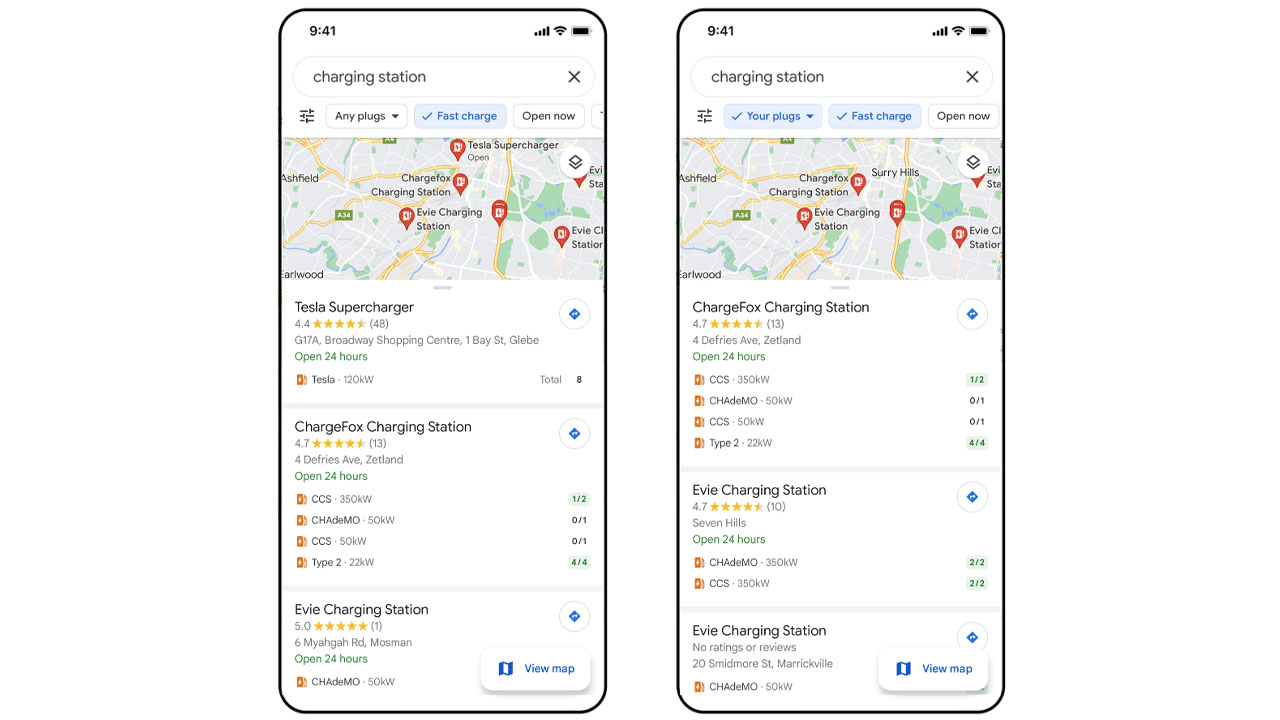The image is split into two sections, each representing a different screenshot of a phone interface. 

**Left Image:**
- At the top right, icons for battery, Wi-Fi, and phone signal are displayed, all filled to the maximum. 
- The top left shows the current time of the screenshot, 9:41 AM.
- Below that, a search bar is visible with the text "charging station," accompanied by an 'X' on the right side to clear the search.
- The categories listed are: "any plugs," "fast charge," and "open now."
- The map features several charging locations plotted, such as "charging station," "Chargefox," "EV charging station," and "Tesla Supercharger." The map view is slightly shifted to the left.
- Below the map, detailed listings include:
  - Tesla Supercharger - 4.4 stars
  - Chargefox Charging Station - 4.7 stars
  - EV Charging Station - 5 stars

**Right Image:**
- Similarly, the top right displays the battery, Wi-Fi, and phone signal icons, all fully filled.
- The current time, 9:41 AM, is shown at the top left.
- The search bar contains the same text, "charging station," with an 'X' on the right side.
- The categories listed here are: "your plugs," "fast charge," and "open now."
- The map presents charging locations, arranged slightly differently, including "charging station," "Chargefox," "EV charging station," and "Tesla Supercharger."
- Below the map, the listings are noted as:
  - Chargefox - 4.7 stars
  - EV Charging Station - 4.7 stars
  - EV Charging Station - no reviews yet

Both images have a similar interface with slight variations in map positioning and order of charging stations listed.